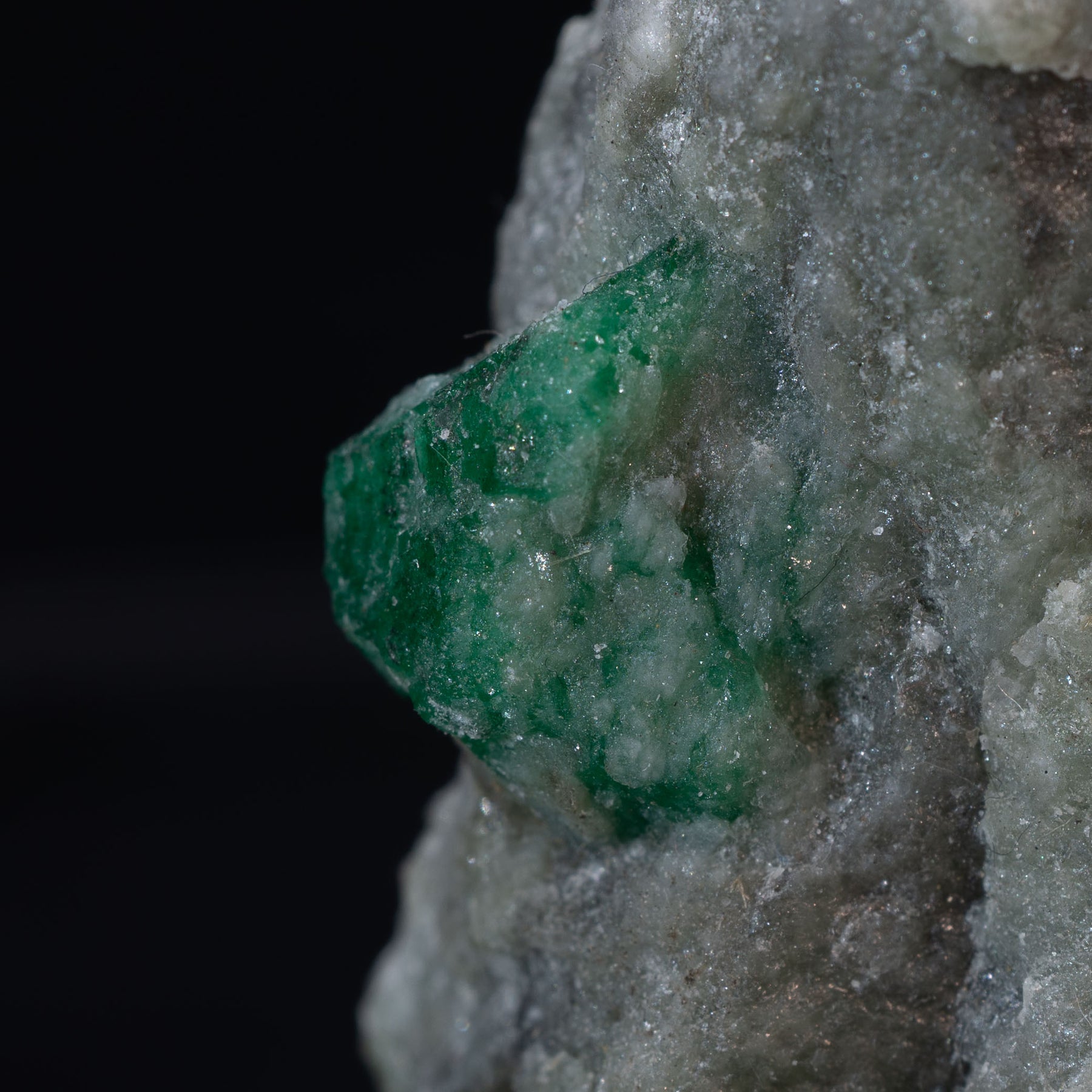This is a detailed close-up of a unique rock formation against a black background. The main feature is a striking green gem embedded in a gray and white rock. The rough, white crystal formations on the rock give it a glistening, almost wet appearance, with a bubbly texture in some places. The green gem emerges prominently from the rock, jutting out in a distinctive triangular shape, dotted with white and gray spots. The rock itself extends from the right-hand side of the image, taking up a significant portion of the frame, with the left side remaining predominantly black.